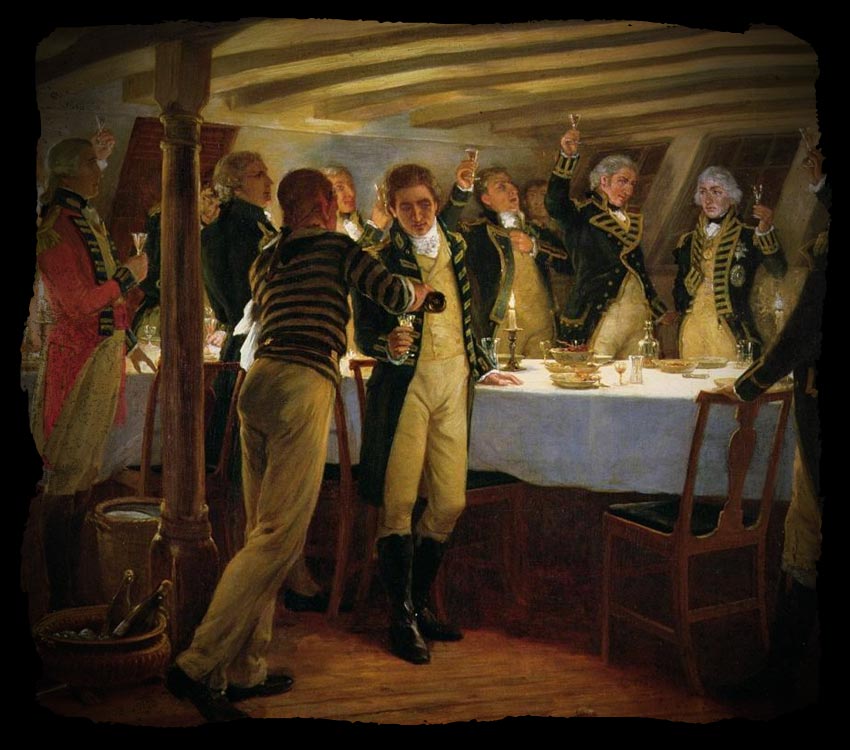This image is a detailed fragment of a painting depicting a gathering of military officers inside an old sailing ship’s interior. The compact room has a low wooden ceiling with closely positioned slats and a wooden floor. At the center, there is an oval-shaped banquet table covered with a white cloth and illuminated by a few candles. The table is adorned with various dishes, cutlery, and several bottles, possibly containing wine or champagne.

The room is filled with uniformed officers, most of whom are wearing blue coats adorned with gold or yellow stitching and black lapels, paired with white pants and black boots. All the men present are standing around the table, engaged in what appears to be a celebratory toast, with glasses raised high in the air. Among them, a distinct figure in a red jacket stands out, possibly denoting his higher rank.

In the foreground, a man with his back turned to the viewer wears a black and white striped shirt with white pants. He appears to be serving alcohol from a large pot filled with bottles to another officer who faces the viewer. Some officers also sport white wigs, adding to the old-fashioned military ambiance of the scene. The painting, bordered by black and seemingly torn at the edges, captures a moment of camaraderie and celebration among the ship’s officers.